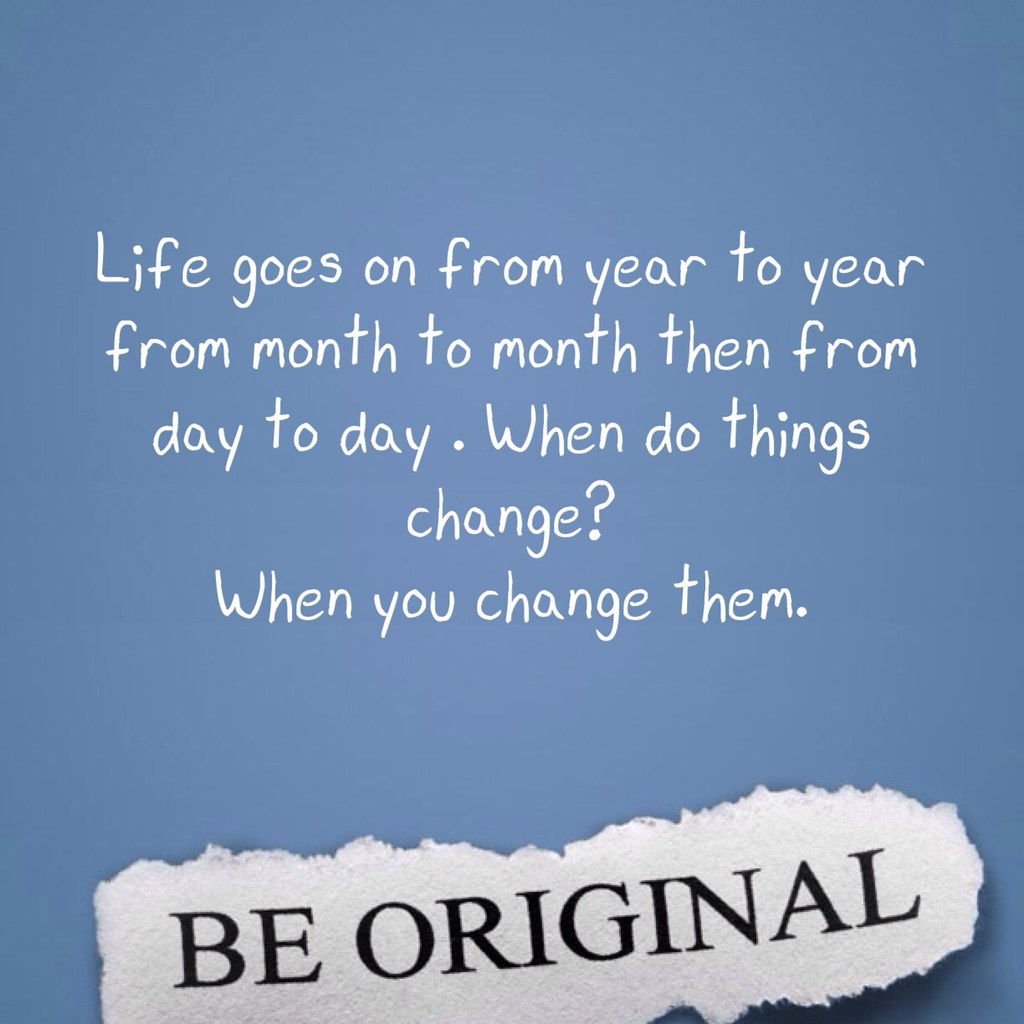The image is a visually striking inspirational poster set within a square frame. The background is a rich, deep blue, reminiscent of a night sky, creating a calming yet poignant atmosphere. At the center of this blue expanse, five lines of white text, styled in a handwritten-like font, deliver an uplifting message: "Life goes on from year to year, from month to month, then from day to day. When do things change? When you change them." Below this motivating quotation, there's an element that uniquely stands out—a small, torn piece of white paper placed within the image, bearing the bold, all-uppercase directive "BE ORIGINAL" in black text. This distinct detail adds a layer of originality and encourages individuality, further enhancing the inspirational theme of the poster.